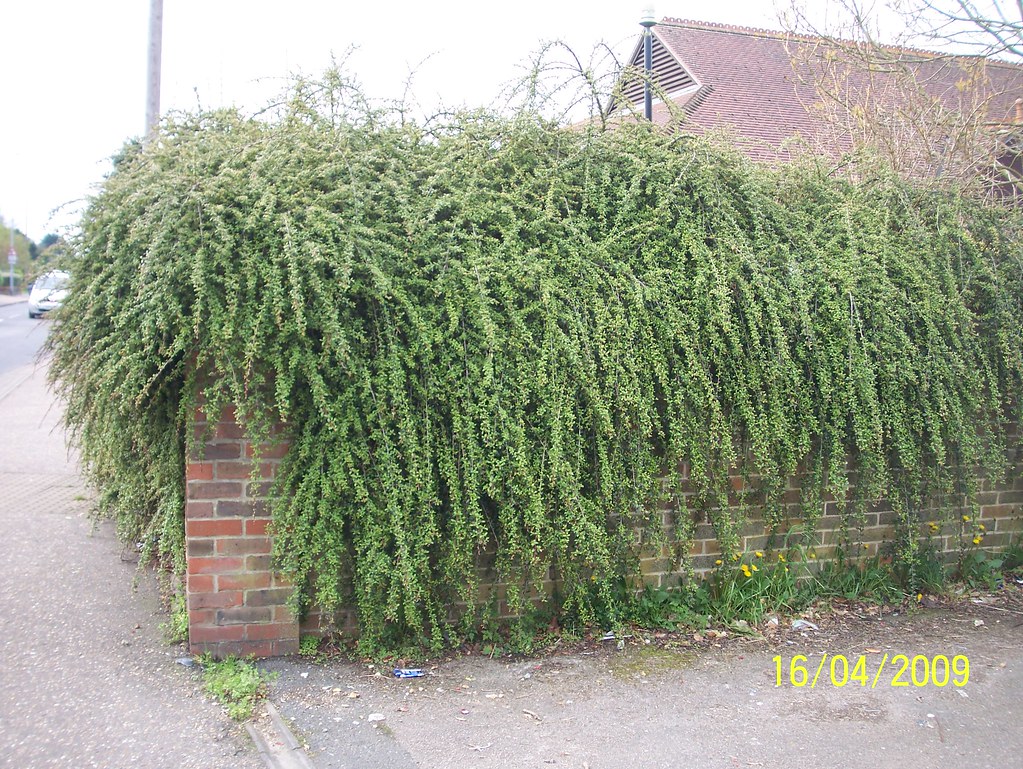The photograph, dated 16-04-2009 in the bottom right corner, depicts a heavily overgrown landscaping plant known as the Cotton Easter draping over the corner of a red brick wall. The Cascade of dusty green leaves and stems nearly reaches the dark concrete sidewalk below, which curves around this street corner. Clusters of vines and fine, delicate stems densely packed with tiny green leaves cover the brick wall almost entirely. At the base of the wall, about ten bright yellow dandelions bloom amidst some discarded rubbish, including a can. In the background, the peak and tiled roof of a house are visible, along with a car parked on the nearby street. The overall scene conveys a lush, albeit slightly unkempt, urban landscape.